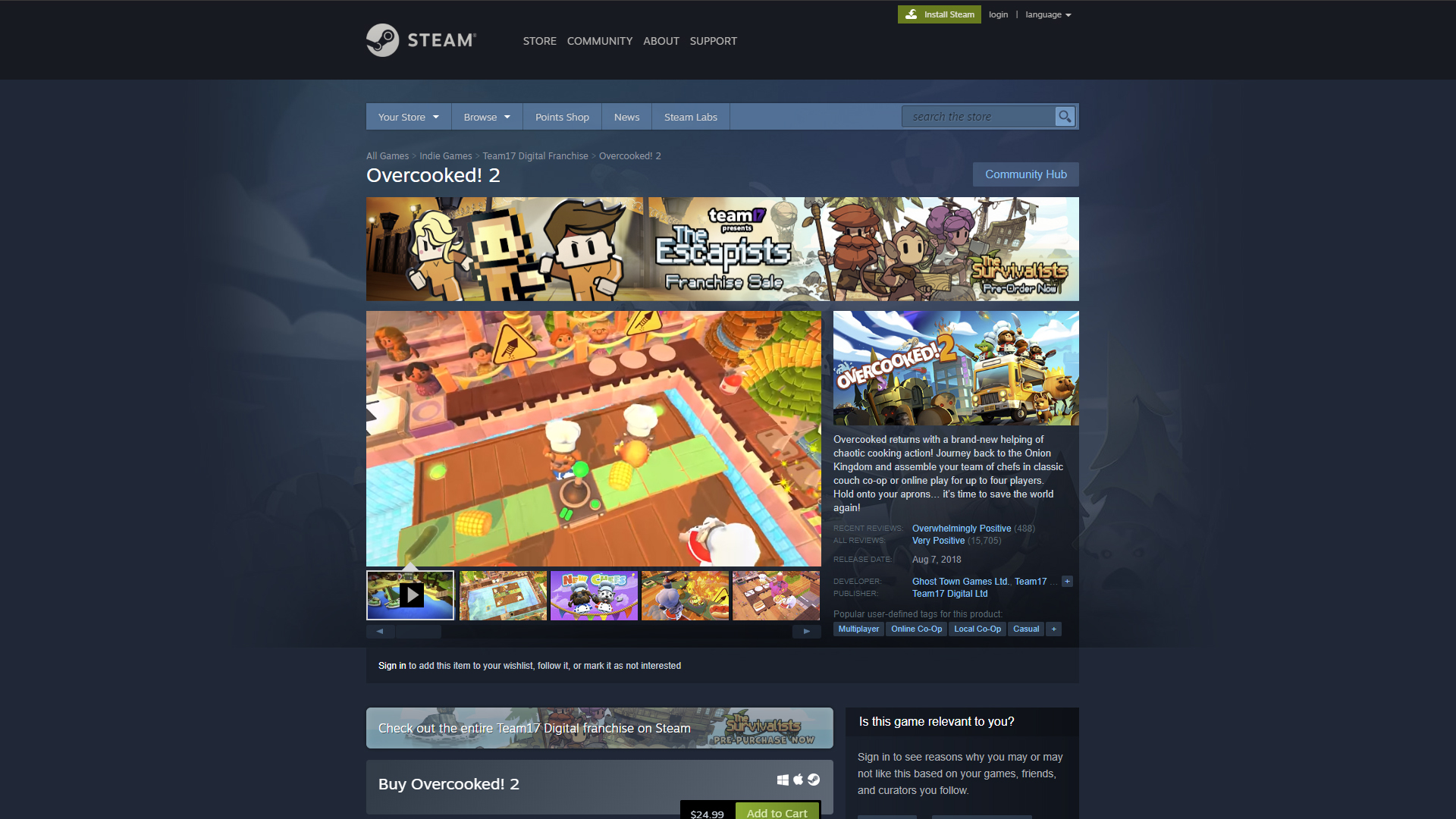On the webpage, dedicated to online game distribution, the main theme is showcased prominently. The spotlight is on the game "Overcooked 2". A banner at the top announces, "Team P presents the Escapists Franchise Sale". To the left, there are illustrated characters from the Escapists series. Nearby, a separate image features three characters from "The Survivalists". The centerpiece of the page is a large, albeit low-resolution, image depicting "Overcooked 2" in a third-person perspective, possibly at a buffet scene. The specifics of the image are unclear due to the resolution. Below this main image, the call-to-action reads "Buy Overcooked 2", accompanied by an "Add to Cart" button. The price, however, is illegible.